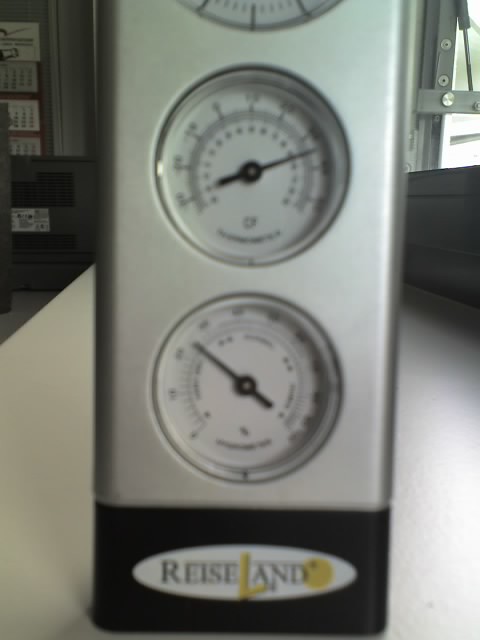The photograph features a precise measuring device with a sleek, stainless steel rectangular body, resting on a pristine white table. Embedded within the stainless steel are two circular dials, each with a crisp white face. The dials are marked with clear black text and numbers, and each has a single black pointer to indicate measurements. The exact function of the dials is ambiguous; they might be measuring temperature, humidity, or possibly speed. Below these dials, the device showcases a distinctive black strip, which is adorned with an oval white section. Within this white oval, the text "R.E.I.S.E.L.A.N.D." is prominently displayed. The meticulous design and thoughtful layout of the components suggest a tool built for accuracy and reliability.